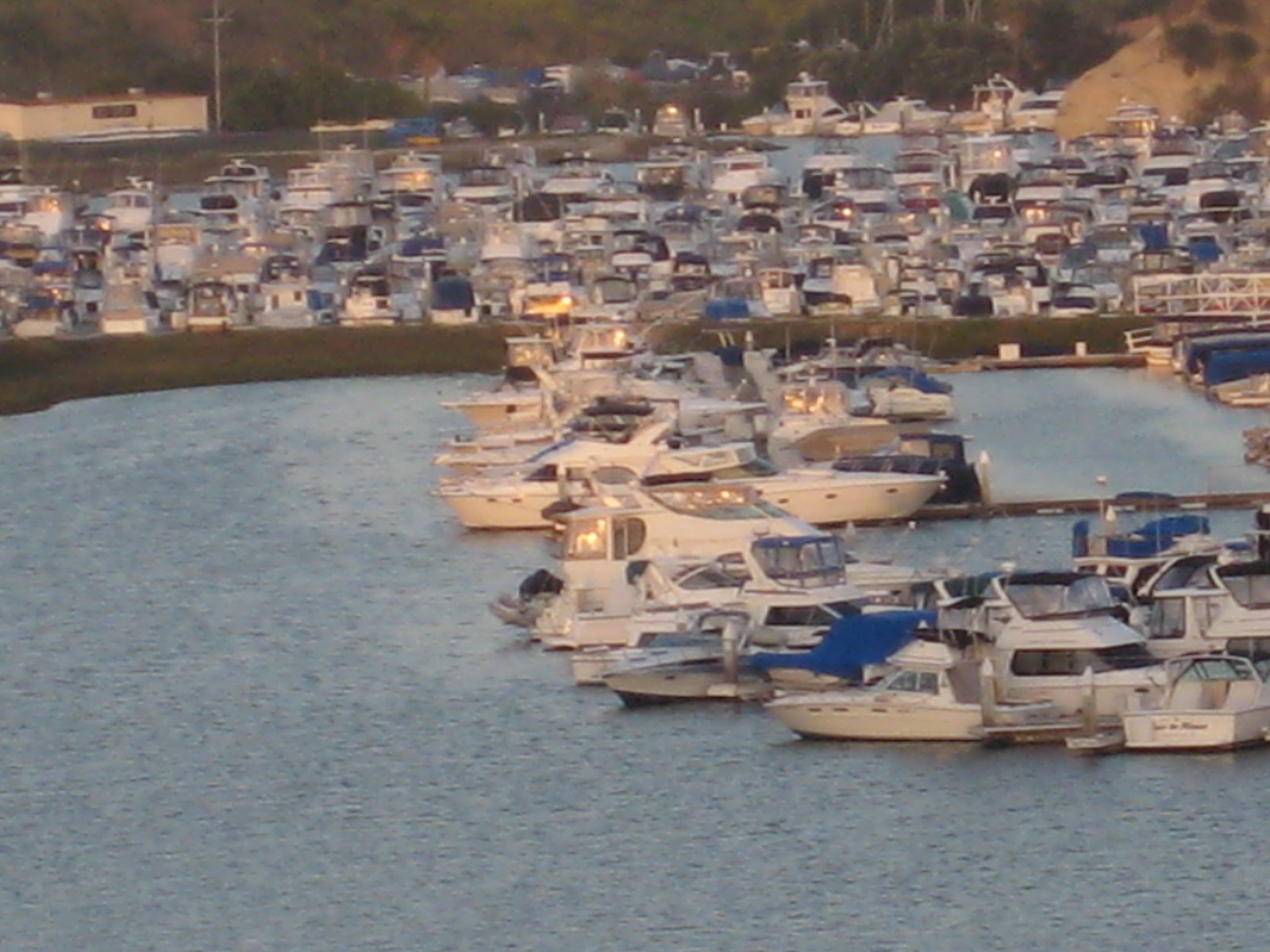This photograph, taken outdoors at dusk, captures a bustling marina or yacht club, likely situated along a lake, river, or dam. In the top half of the image, the water area is packed with numerous small boats, many of which have their lights on, signifying the approach of nightfall. Separated by a prominent brown or concrete barrier, the front area of water contains fewer boats, about 10 to 12, compared to over 30 boats densely packed in the background. These boats, predominantly white with some featuring blue covers, also have interior lights illuminated. Along the barrier, there appears to be a stretch of land with soil and grass, extending horizontally across the middle of the scene. In the far background, a few buildings or houses, possibly part of a small community, are visible, surrounded by trees and set against the backdrop of a distant mountain range. The serene blue waters enhance the tranquil yet lively atmosphere of this marina at dusk.